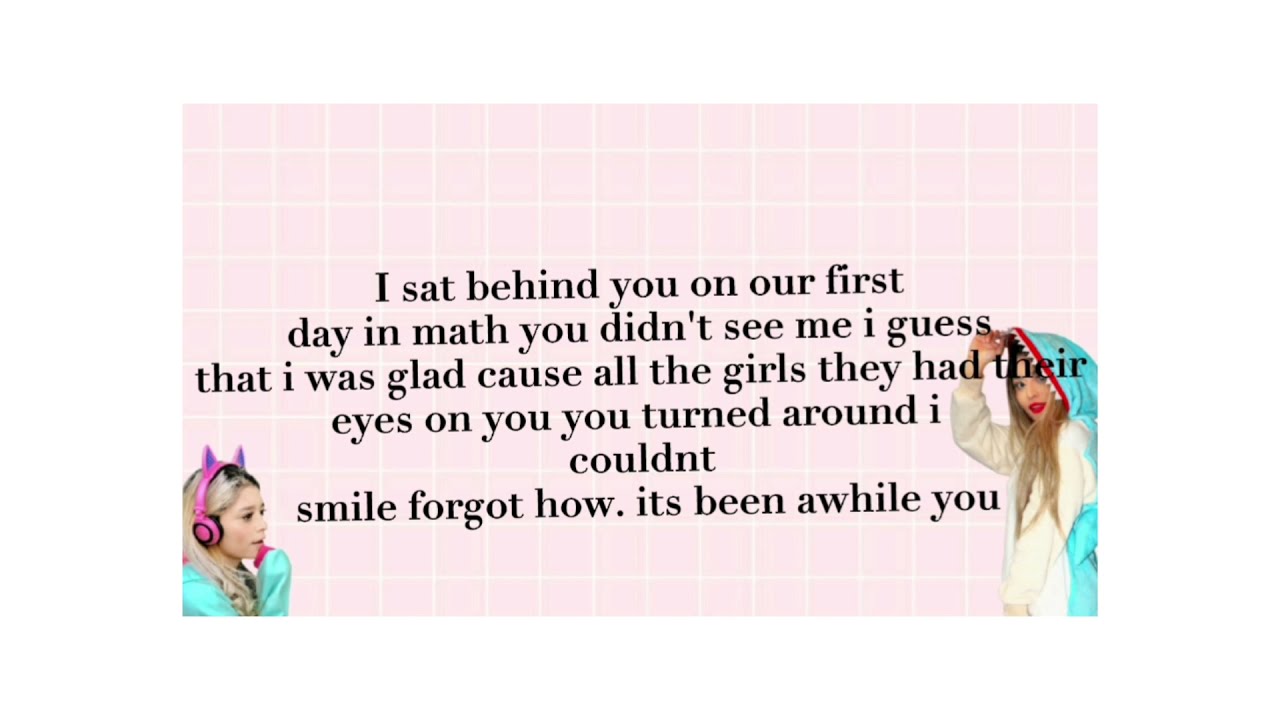The image features a pink background with white grout lines creating a checkerboard pattern of small pink tiles. Centered on this background is a black text message that reads: "I sat behind you on our first day in math. You didn't see me, I guess, and I was glad because all the girls had their eyes on you. You turned around and I couldn't smile, forgot how. It's been a while, you." In the lower left corner, a white girl with blonde hair pulled back, wearing a green shirt and pink headphones with cat ears, gazes across the image. In the lower right corner, another white girl with long blonde hair, red lipstick, and a white shirt is dressed in a teal shark hoodie, her hand resting on the top where the shark's teeth are visible.